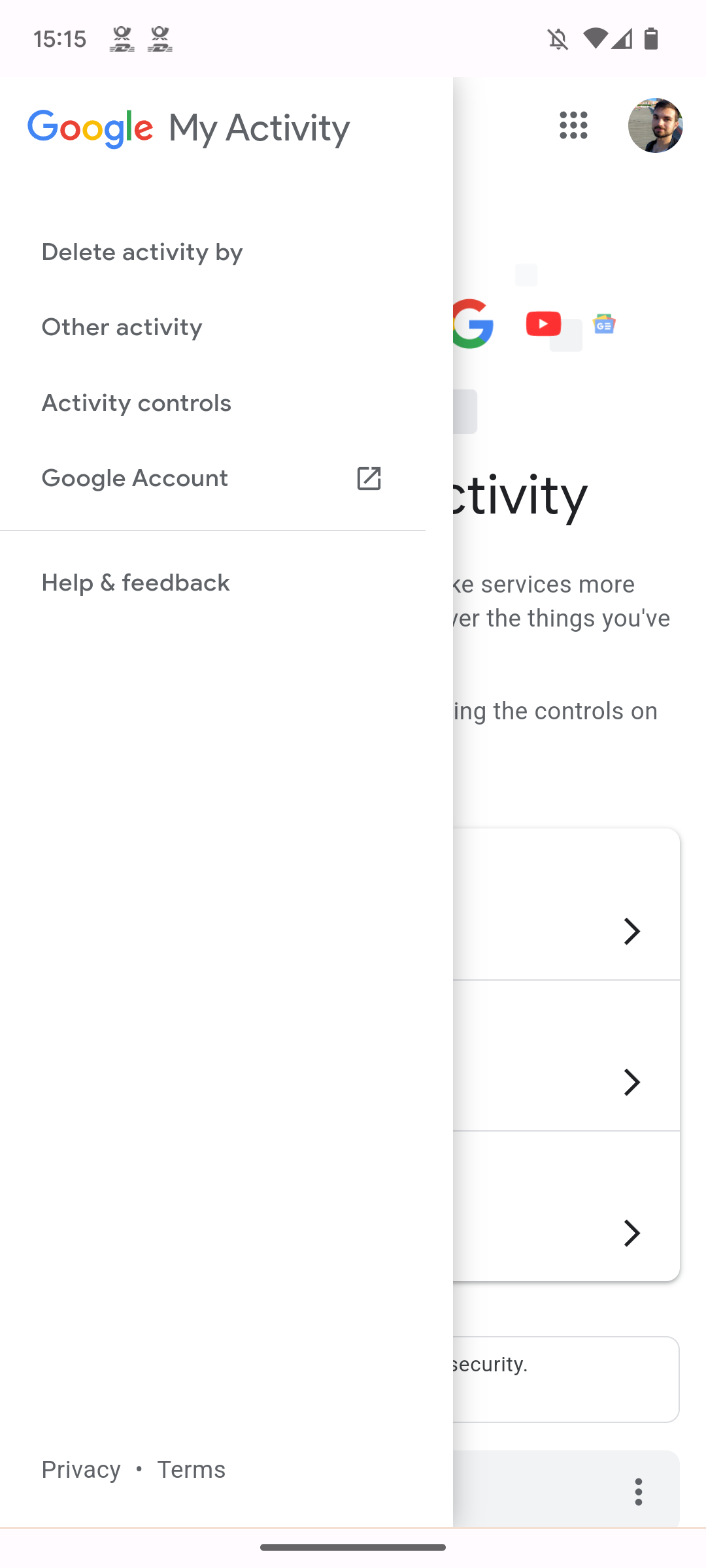This image appears to be a screen capture of a smartphone displaying a Google My Activity page, which partially overlaps another screen in the background. The primary focus of the image is the top screen, where the Google logo is prominently displayed in its signature multi-colored font, followed by the text "My Activity" in plain black letters. 

At the very top of the screen, the time is displayed as "15:15." Below this, the main content of the Google My Activity page lists several options: "Delete Activity By," "Other Activity," "Activity Controls," "Google Account," a faint gray separator line, and finally "Help and Feedback."

On the right side of the image, the overlapped screen from the background becomes visible. There is a partially transparent profile picture of a man with dark brown hair, dark eyes and eyebrows, a mustache, and a small beard. The profile picture is circular, and underneath it, part of the word "Activity" is visible, truncated to "Civity."

The composition of the image, with the layered screens and the detailed elements in the interface, captures a snapshot of the Google My Activity page in use.